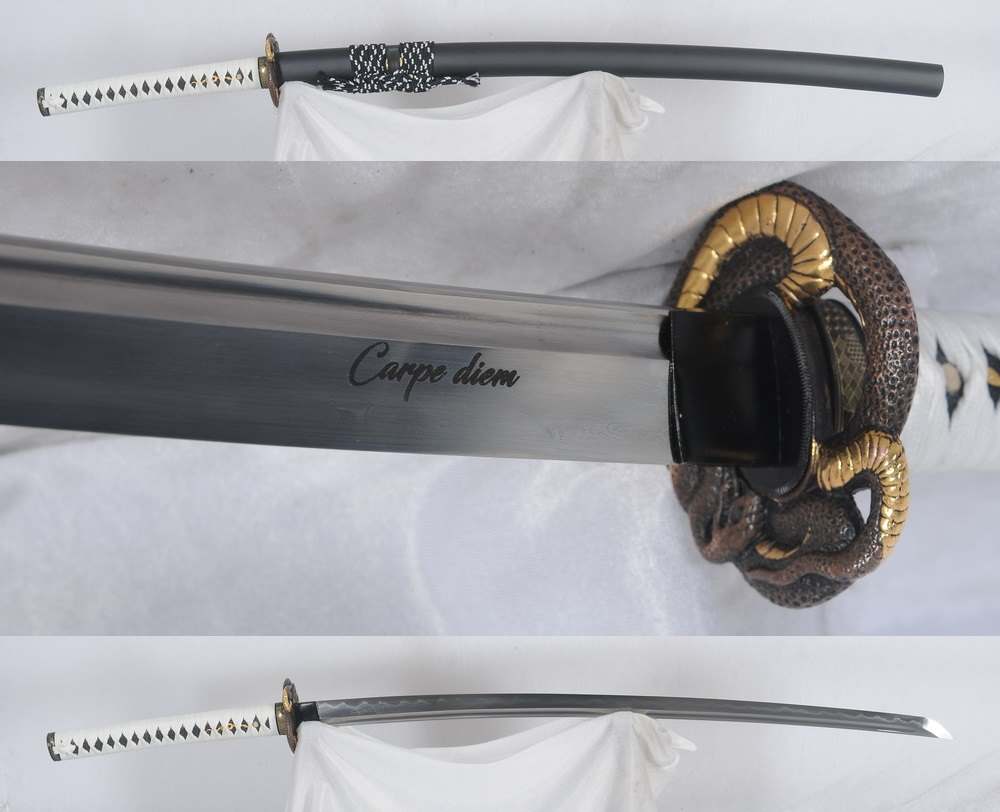The detailed image showcases a samurai sword in three distinct panels, each providing a different perspective. The top panel features the sword resting in its gray scabbard, displayed on a stand draped in elegant white fabric against a white wall. The handle is visibly wrapped in white leather, and the scabbard is secured with a black and white tie. The middle panel offers a closer look at the blade, revealing the engraving "Carpe Diem" in cursive writing. This panel also highlights the ornate hilt, intricately designed with gold and brown snake-like patterns. Finally, the bottom panel displays the fully unsheathed silver sword lying on the same fabric-draped stand. The composition of the three images is intended to emphasize the sword’s craftsmanship, elegance, and striking potential.